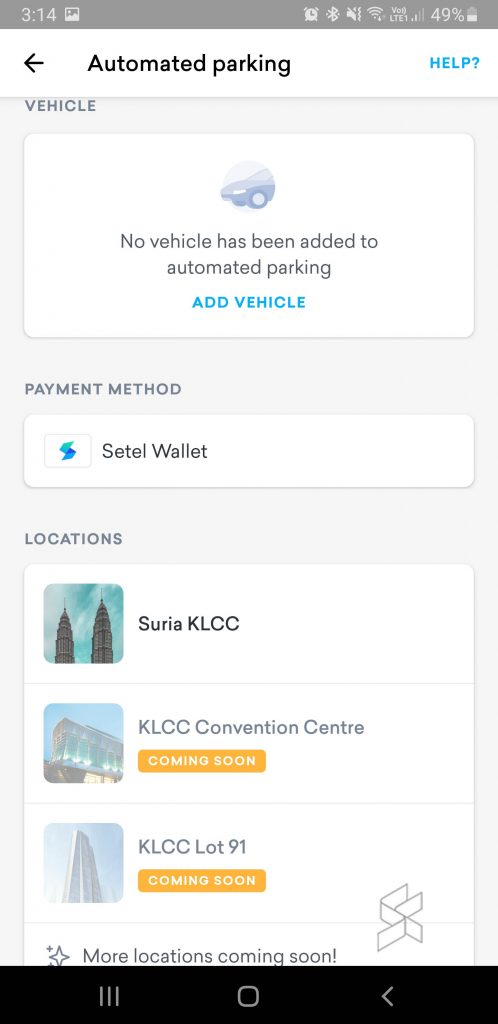The image displays a graphical interface of a cell phone screen featuring a parking application. At the top of the screen, bold blue capital letters spell out "AUTOMATED PARKING", accompanied by a question mark icon situated to its right. Below this, the user interface presents a section titled "Vehicle", which contains a white rectangular field indicating that no vehicles have been added to the automated parking system. Beneath this, in prominent blue capital letters, there is an option labeled "ADD VEHICLE."

Further down, the interface includes a section for "Payment Method," within which a white rectangular field shows "SETEL Wallet." Next, the "Locations" section showcases a series of entries with corresponding images and descriptions. The first entry features an image of two towers, labeled "SURIA KLCC." Below this entry, another image denotes "KLCC Convention Center," and a yellow rectangle beneath it is marked "COMING SOON." Following this, another entry named "KLCC Lot 91" similarly features a "COMING SOON" notice.

Overall, the displayed parking app indicates that no vehicles have yet been added, one location is active, and two additional locations are forthcoming.